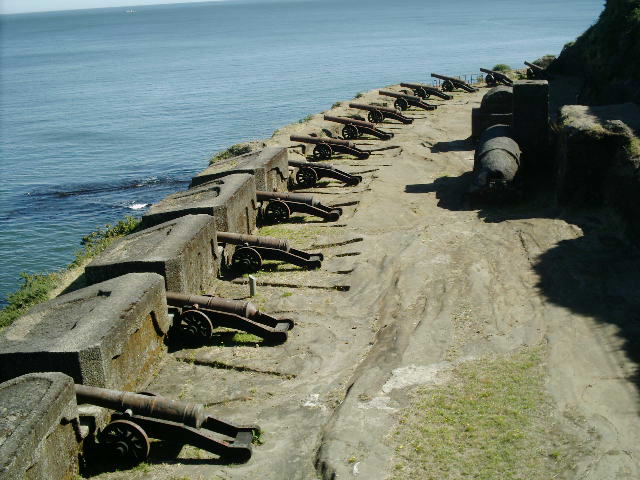The image depicts a serene scene of an old fort situated on the edge of an island or seashore. The top left corner of the photograph showcases a calm, dark blue ocean, with a white boat visible in the distance. The fort itself features a semi-circular arrangement of 14 rusted, brass-colored cannons, each positioned within concrete cutouts along the wall, all aiming towards the ocean. The ground within the fort is a mix of rocky brown terrain and patches of grass, with a gravel road interspersed with some greenery running directly behind the cannons. Additionally, there is a large round structure on the far side of the road, partially obscured but adjacent to a rising steep hill. The photograph, taken from a slightly elevated perspective, emphasizes the fort's strategic placement and historical significance.